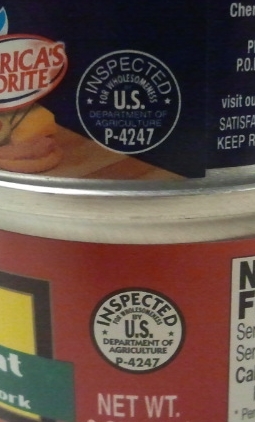This close-up photograph features part of a food container with various detailed labels and stickers. At the top, there is a white oval with red lettering that partially reads "Rica's Rite." Directly below, a white-bordered round sticker prominently displays "Inspected U.S. P-4247." Below this sticker, there's a silver or metal rim separating the top section from a red lower section, which also contains another circular sticker stating "Inspected by U.S. Department of Agriculture, P-4247." On the right side of this red section, there is an unreadable white label with black lettering that is cut off. To the left, there is a green section with more illegible writing. Additionally, the red part of the container includes more stickers: a white circle with black text indicating inspection details, further affirming the presence of the U.S. Department of Agriculture marks. The image includes other stickers with various designs, including one in the bottom-left with a yellow background and green text, and another on the right showing a white sticker with cut-off black text. A distinctive red logo with blue lines and white areas also appears on the left side of the top section, along with other partially visible colorful elements, including yellow and pink images.